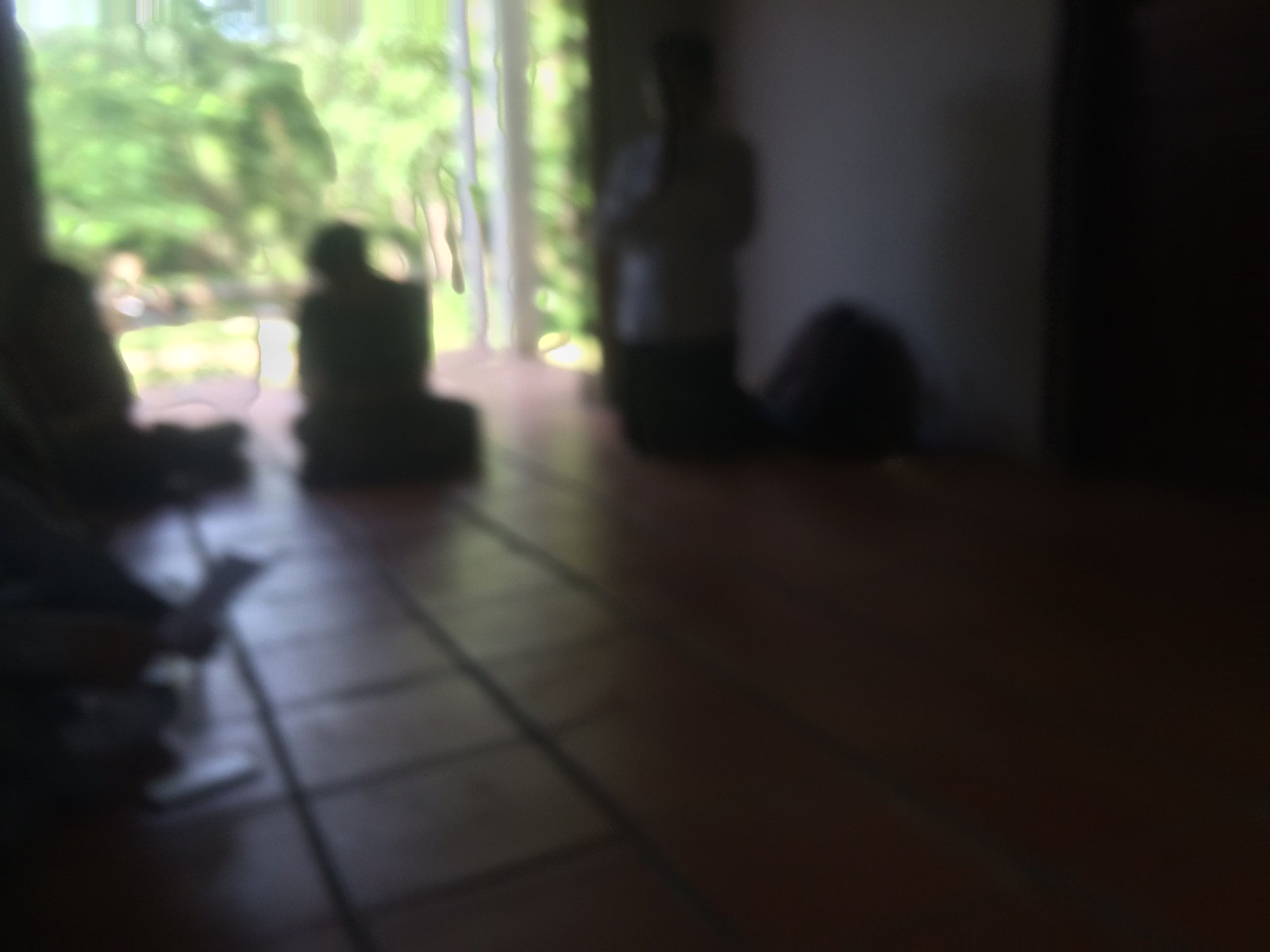The image depicts an out-of-focus scene of an open hallway leading to an outdoor area. The hallway is adorned with possibly brown tile flooring. Along the left-hand side, there appear to be at least two people, while the right side has at least one visible figure. Despite the blur, the hallway's opening reveals a hint of greenery, potentially grass, with a mix of light and yellow-green hues. In the far background, trees can be faintly discerned. A structural support pole is vaguely visible within the hallway, adding to the overall sense of depth. The image is overall quite dark, adding to the obscurity and indistinct features.